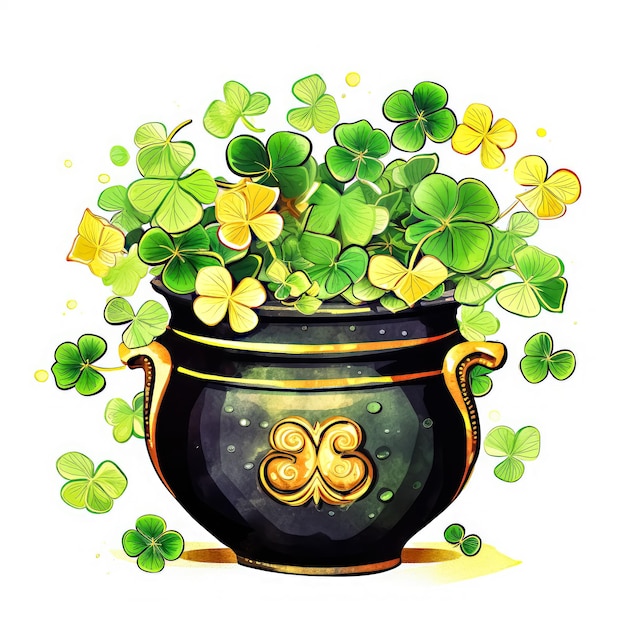This image is an artist's hand-drawn or AI-rendered illustration set against a white background. It features an elegant, predominantly black vase adorned with intricate gold details. The vase has gold rings around the top, gold handles on the sides, and a prominent gold emblem on the front, which some have speculated might resemble a butterfly. The base of the vase is also trimmed in gold, giving it a refined and luxurious appearance. This elegant pot is overflowing with a chaotic array of clover, mostly four-leaf clovers, but some three-leaf clovers are also present. These clovers vary in color, from lighter yellow greens to more traditional dark greens. The clovers are irregularly shaped and crammed into the vase, with several spilling out and drifting gently to the surface below, emphasizing the abundance and almost whimsical nature of the illustration.